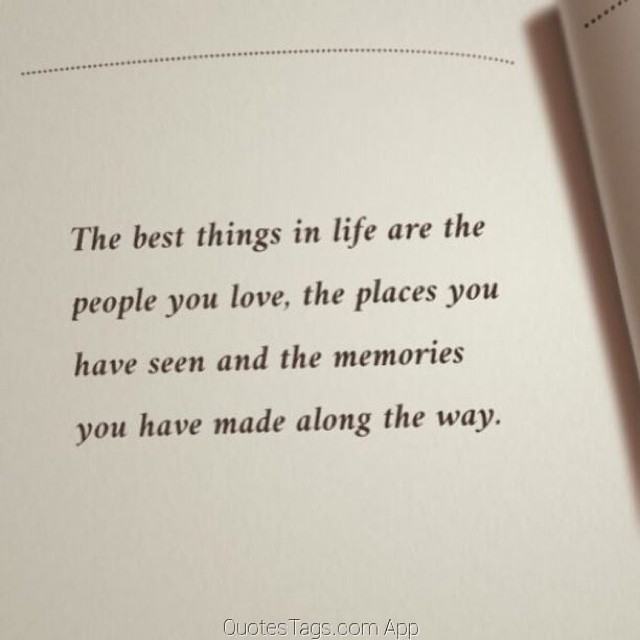The photograph captures an up-close view of a cream-colored page from an open book. Along the top of the page, a decorative border of tiny black dots is visible. Centered both vertically and horizontally on the page is a passage written in announcement style lettering: "The best things in life are the people you love, the places you have seen, and the memories you have made along the way." Below this text, in light gray with a subtle black drop shadow, is the text "QuotesTags.com App." To the right, the partially folded next page casts a soft shadow on the left side of the open book, adding depth to the image.